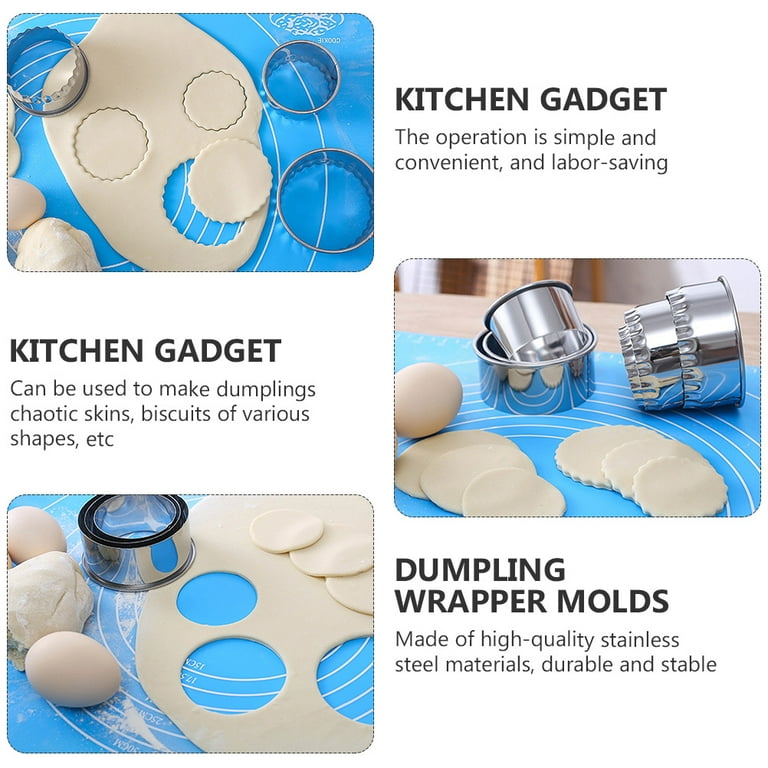This is a detailed advertisement image for a set of kitchen gadgets, which includes three circular stainless steel molds of varying sizes. The layout is organized with both images and text in different sections. 

**Top Section:** On the left side, there's a photo featuring an oval sheet of rolled-out dough on a blue baking mat, which has white measurement rings for size reference. The dough has been cut using ridged circular molds, leaving three distinct impressions. One of these cut-outs is partially removed, demonstrating ease of use. To the right, text reads: "Kitchen Gadget. The operation is simple and convenient and labor-saving."

**Middle Section:** Text on the left explains further uses: "Kitchen Gadget can be used to make dumplings, chaotic skins, biscuits of various shapes, etc." On the right, there's an image showing the various sizes of cut-out dough pieces stacked in a pile or lined up near a ball of dough, emphasizing versatility and efficiency.

**Bottom Section:** On the left, an image displays smooth-edged circular molds and dough pieces, some rolled up like dumplings. Next to this, the text declares, "Dumpling wrapper molds made of high-quality stainless steel material, durable and stable." The layout and captions clearly illustrate that these durable kitchen tools simplify dough cutting tasks, making them perfect for a variety of culinary applications.

All the text is in black lettering, complementing the professional look of the advertisement.